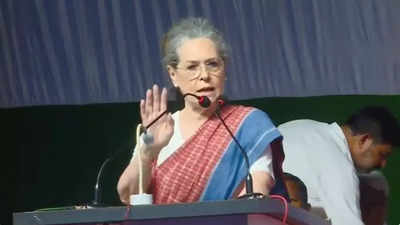In this photograph, an older woman with gray hair pulled back into a bun stands at a podium, giving a speech. She speaks into two microphones, one on a white base and one on a black base, with her right hand raised as if to emphasize a point or signal for attention. She wears wire-rim glasses and a white short-sleeve t-shirt, over which drapes a traditional Indian sari that is red checkered with a blue cambray material hanging over her shoulder. The backdrop behind her is a mix of hunter green and pleated blue fabric, providing a professional setting. To her right, slightly behind her, a man with black hair and a mustache, dressed in a long-sleeve white shirt, is bent over as if picking something up. Additionally, just visible in the corner of the image, the top of a small child's head and eye can be seen.